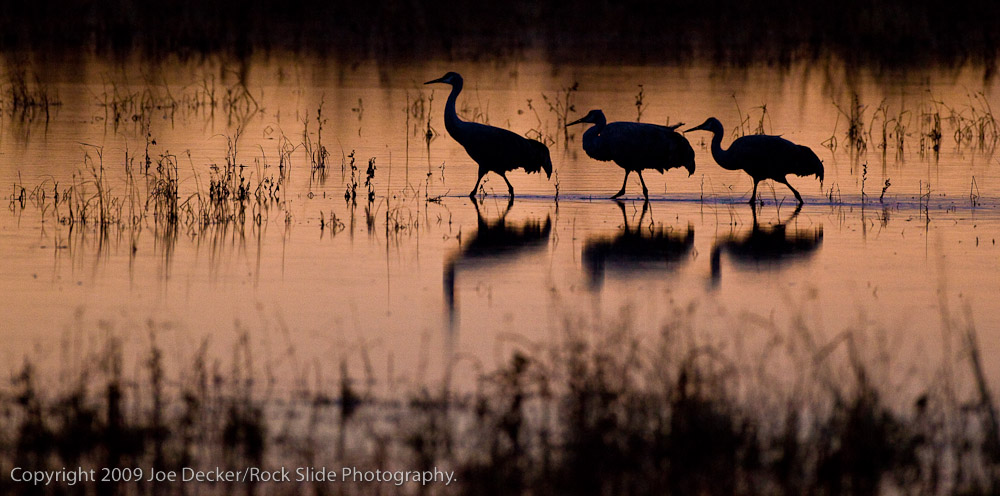This landscape photograph, approximately twice as wide as it is tall, captures a serene, shallow marsh or pond at sunset. The bottom left corner features the text "Copyright 2009 Joe Decker / Rock Slide Photography." Dominating the scene is a marshy water body tinged in a captivating pink hue, bisected by a thin line of blue where three tall birds, likely cranes, wade gracefully. Their dark silhouettes stand out against the colorful backdrop: the first bird stands with its neck outstretched upward, while the second bird has its head tucked into its neck, and the third bird has its head lowered but not fully crouched. Delicate plants and reeds emerge from the water, adding to the tranquil ambiance. The photograph's top and bottom edges dissolve into shadowy black, further emphasizing the rich, sunset colors and the elegant reflections of the birds in the water.